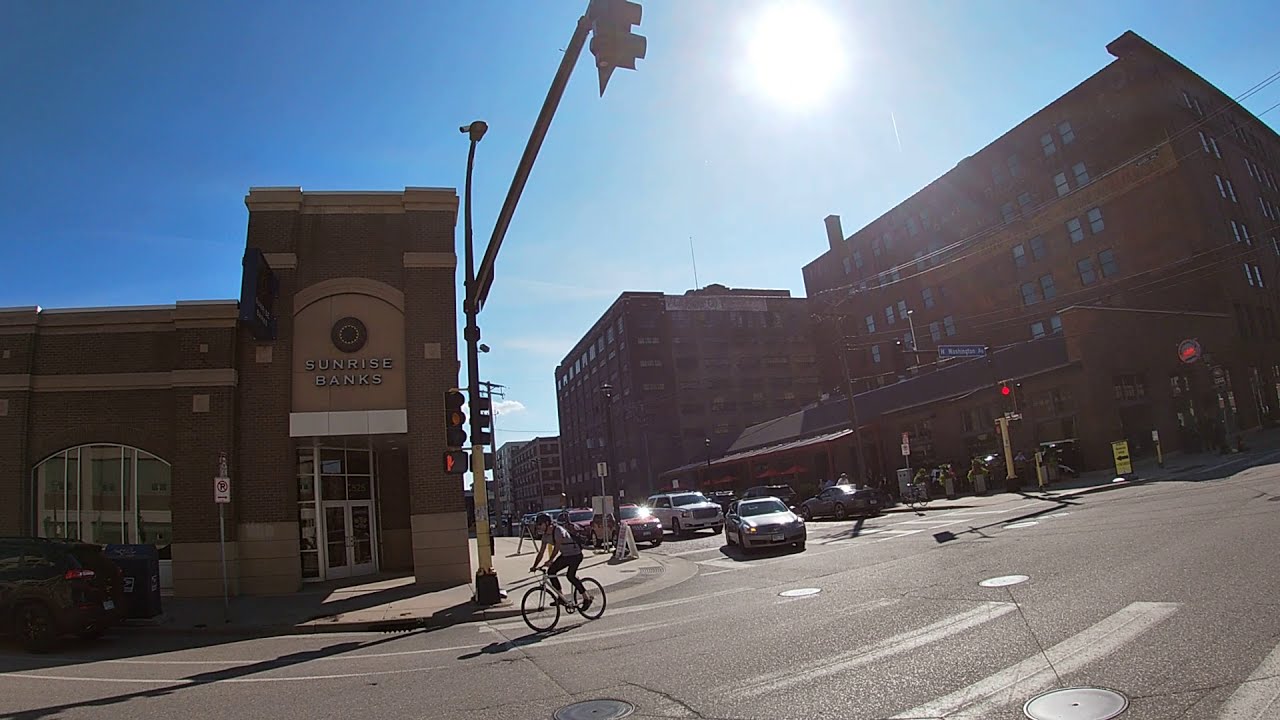This detailed photograph captures a bustling downtown district during a sunny summer afternoon. We are positioned at a four-corner intersection, with the paved streets clearly marked by white crosswalk stripes. The scene is alive with activity; cars wait patiently at the light, both on the street and parked along the side. In the foreground to the left, the Sunrise Bank building stands prominent, displaying its name in white print against its brown facade. A shirtless male cyclist rides his bicycle on the left side of the image, preparing to turn the corner. Tall brick buildings rise at the intersection's right-hand corner, their impressive heights silhouetted against a bright blue sky with just a few clouds. The sun is high, casting a vivid light that accentuates the energy of this urban setting. Streetlights, mounted high, oversee the bustling intersection, adding to the structured yet dynamic cityscape.